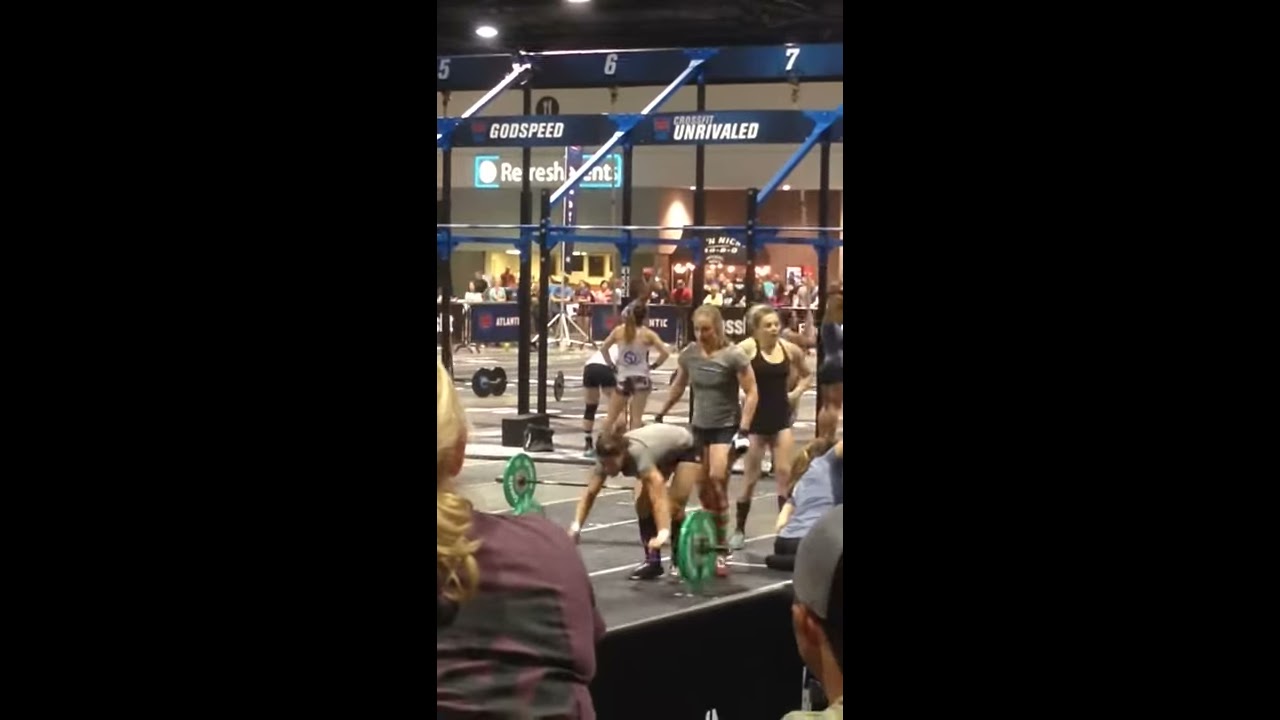In this image taken within a high-ceilinged indoor fitness center, we see what appears to be a women's powerlifting competition. Dominating the center of the photograph, a dark-haired woman dressed in a gray t-shirt, black shorts, and black sneakers is bent over, gripping a pair of green barbells, poised to lift them. Right behind her stands another woman in a similar gray t-shirt and black shorts, with blonde hair. Further back, another blonde woman dressed in a black tank top is positioned with her hands on her hips, observing the scene. 

In the foreground on the left, the shoulder of yet another blonde woman can be seen, indicating she is also watching the action. The background reveals a panel of judges seated at a large table beyond a metal and glass partition, with several more women in identical gray and black outfits standing with their backs to the camera, facing the judges. Above this assembly, a series of banners are displayed: one reads "Refresh Hunt," another has the words "Good Speed" and "Unrivaled," and a third features the numbers 5, 6, and 7, which may denote different competition stations. The scene is vibrant with athletic activity and spectatorship, underscoring the event's organized and competitive nature.